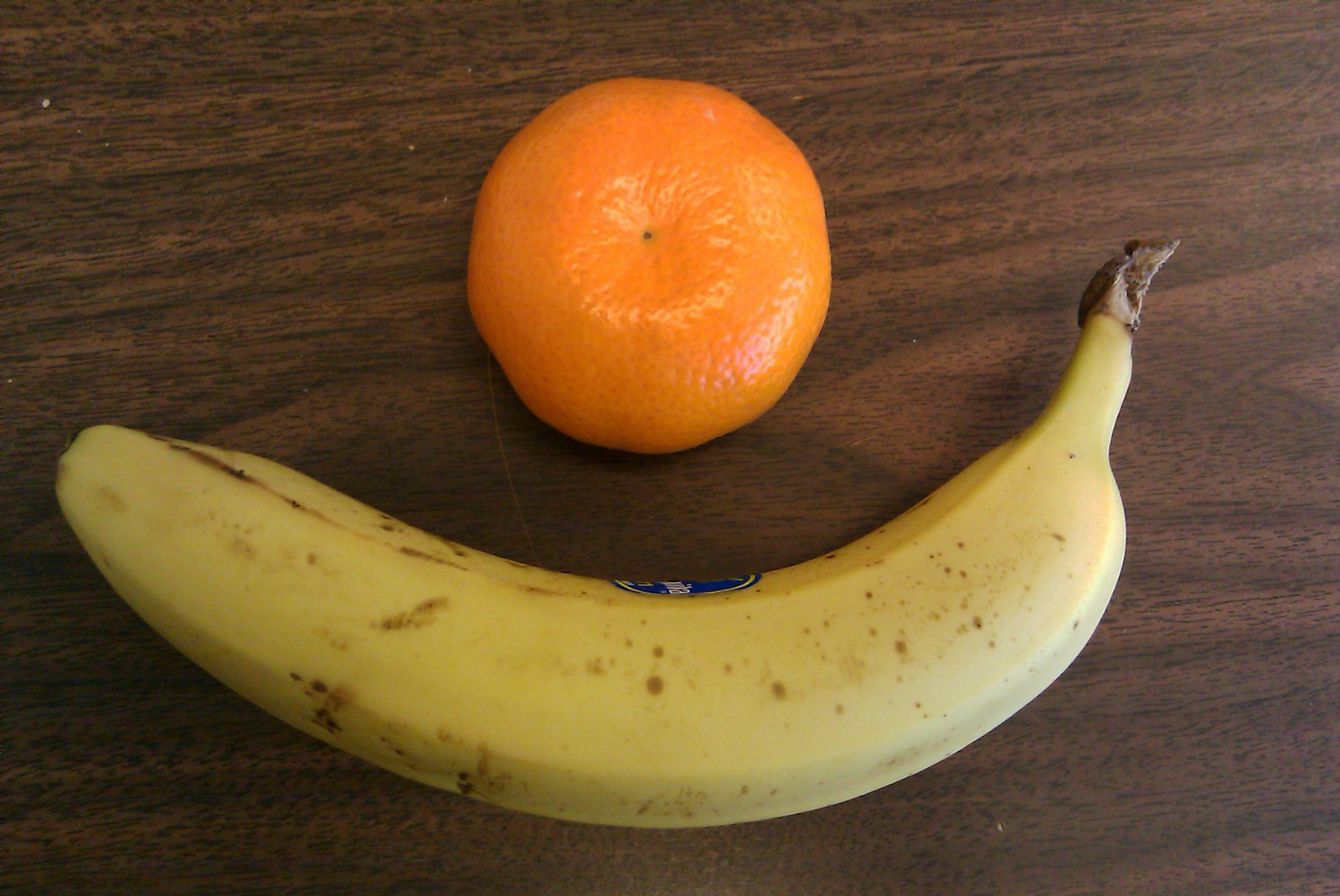In this close-up, top-down shot, a ripe yellow banana rests in a U-shape at the bottom of a dark wood grain table. The banana features a blue Chiquita label and has small black spots, indicating ripeness. Its stem, located on the right, is a darkened brown. Sitting in the middle of the banana's curve is an orange or tangerine, identifiable by a distinct black dot at its center. The dark wood grain background on both the left and right sides adds a rustic touch to the composition.